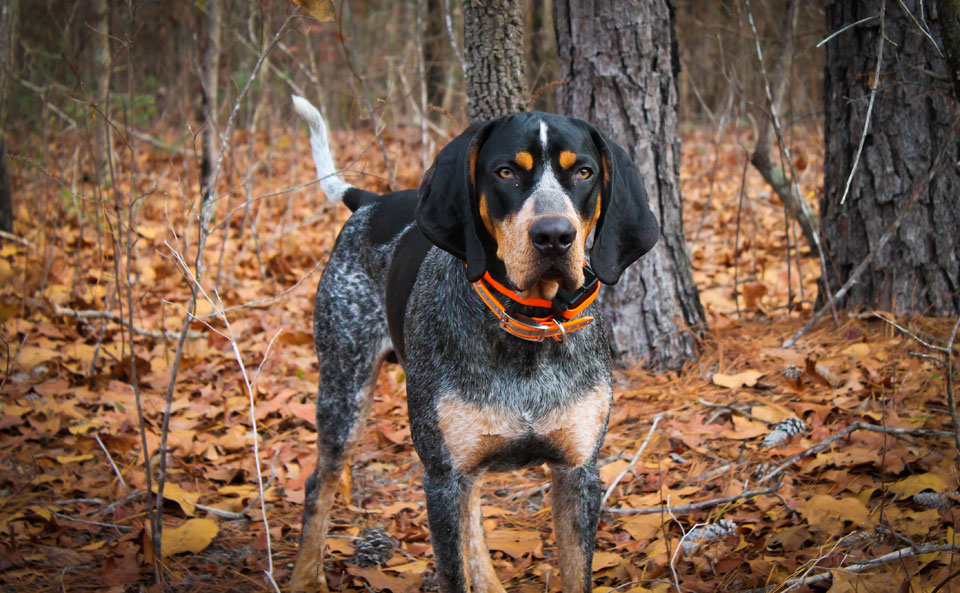In a serene autumn forest, amidst a carpet of vibrant orange and brown leaves, stands a medium-sized, multi-colored dog, exuding both attentiveness and grace. The dog, predominantly black with streaks of white and splashes of brown, showcases an intricate mix of colors: black floppy ears frame its face, and its white-tipped tail contrasts against its darker body. Brown patches accentuate its legs, lower chest, and parts of its face. Adorning the dog is an orange collar, possibly layered with another, hinting at the possibility of this being a hunting or working dog. With a serious and focused gaze directed just off the side of the camera, the scene suggests a moment of alertness or readiness, perfectly harmonized with the backdrop of barren tree trunks and fallen autumn leaves.